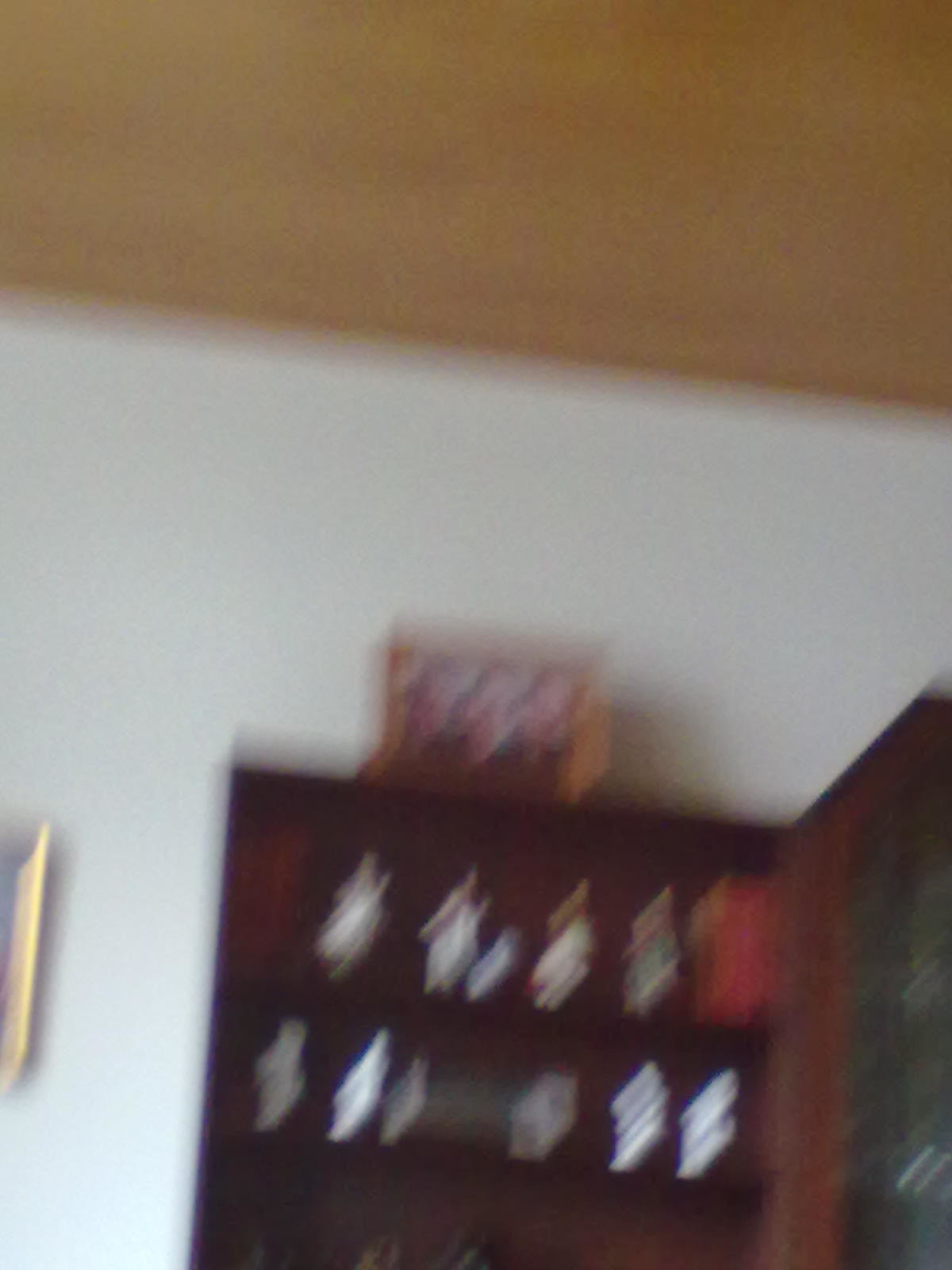This photograph captures a slightly blurred interior wall, likely within a home. The predominantly white wall features a brown band at the ceiling's edge. Positioned against the wall is what seems to be a bookshelf or buffet, though its details are obscured by the blur. Atop this piece of furniture sits a framed photograph that appears to depict a family or group of people. Two shelves are visible below, each adorned with unidentified figurines. The image also includes a glimpse of another picture mounted on the wall to the left, housed in a gold frame, though the actual picture within the frame is not visible due to the edge cutoff. The photo is taken from a lower angle, giving a perspective slightly below eye level.